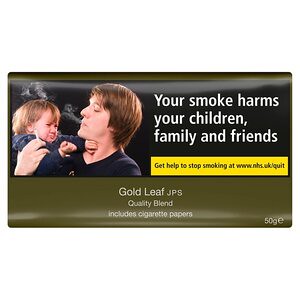In this detailed anti-smoking advertisement, the primary focus is a disturbing scene set against a black backdrop. In the top left corner, a mother is seen holding her baby while blowing cigarette smoke directly into the child's face, causing the baby to grimace and fuss uncomfortably. The advertisement is designed to be striking and colorful, using shades of green, white, yellow, black, grey, brown, tan, and dark blue to grab attention. On the right side of the image, bold white text reads, "Your smoke harms your children, family, and friends." Below this, a yellow bar contains the message, "Get help to stop smoking at www.nhs.uk/quit." At the bottom of the image, the advertisement mentions "Gold Leaf JPS quality blend includes cigarette papers," reinforcing the anti-smoking message by associating it with a known cigarette brand. The entire image effectively conveys the harmful impact of smoking on loved ones, and appears to be a government-issued advisory poster aimed at encouraging smoking cessation.